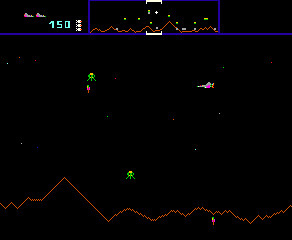The image is a digital screenshot from an older video game, reminiscent of titles from the late 70s or early 80s, and possibly similar to the game Defender. It features a space-like scenario with a dark black background dotted with stars, creating the illusion of outer space. At the bottom of the screen, there is a jagged, orange mountain range, depicted with simple line art. Alien figures, which are green and tentacle-like, are scattered across the scene. A red and white spaceship navigates this environment from the right side of the screen, moving left. In the top right corner, there is a blue "150" score indicator. The top section of the image features a heads-up display (HUD) with two vertical lines forming large squares, containing minimal unreadable text, except for the score. This display gives an overview of the game map and player status, including life count and point tally. Small white missiles appear to be targeting the spaceship from the mountains below.